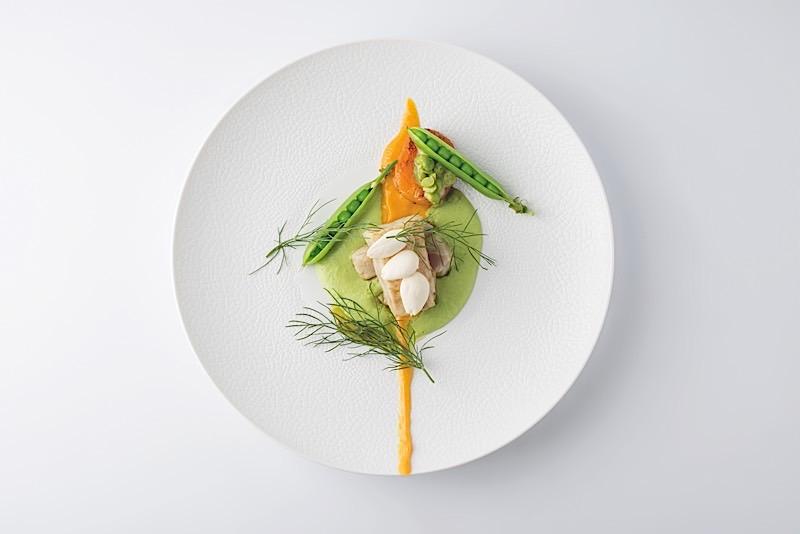The photograph showcases a meticulously presented dish on a white plate, set against a matching white background, emphasizing its elegant presentation. Central to the composition are two pieces of fish arranged in a crisscross or X shape, resting atop a vibrant green wasabi-like sauce. This green puddle extends beneath a thicker line of orange sauce that gradually thins towards the bottom edge of the plate, possibly resembling mustard. Flanking the fish are two open pea pods, each revealing their peas, with one pod nestled on a modest mound of spicy green sauce and the other positioned to the left. The dish is garnished with white bits and tiny plants delicately sprinkled across, adding texture and an upper-end, gourmet appeal. The open pea pods are artistically set at an approximate 90-degree angle from each other, pointing towards the lower left and right corners of the image, creating a sense of balance and symmetry in this expressionist culinary presentation.